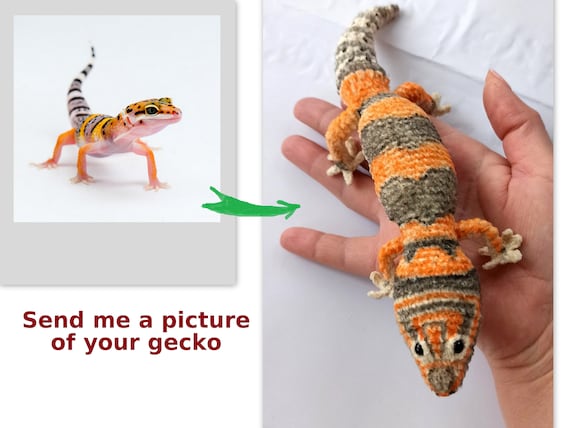This image appears to be an advertisement for a custom service. On the left side, it features a realistic photograph of a gecko with an orange face and legs, a gray and orange striped body, and a tail striped in black, white, and gray. Above this gecko, the text reads, "Send me a picture of your gecko." A green arrow points to the right side of the image, where a person's right hand is holding a handmade replica of the gecko. The replica, possibly crocheted or knitted from soft material like yarn, mimics the original gecko's distinctive colors and patterns, including the orange and gray striped body and the black, white, and gray striped tail. The hand holding the replica gecko has four fingers wrapped around it and the thumb separated, giving the crafted gecko a sense of secure placement and a well-detailed presentation.